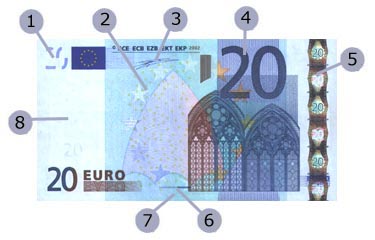The image depicts a detailed diagram of a colorful 20 euro banknote. The banknote is predominantly light blue with accents of white, purple, reddish-brown, and green. The design features a large purple "20" in the center and another "20" on the bottom left. The note showcases three prominent archways in the middle. 

A series of numbered bubbles, labeled 1 through 8, are pointing to various features on the banknote: 
1. The upper left corner pointing to the "20".
2. Surrounding the stars in the middle of the banknote.
3. The top middle section.
4. The upper right corner showing another "20".
5. A strip on the right side of the note containing the numeral "20" and an unspecified figure.
6. The lower right corner,
7. The bottom left,
8. The left edge of the note.

Additionally, the pattern includes green heart-like shapes outlined in white, and there appears to be a column on the right side detailed with a vertical "20". This diagram seems to serve as an explanatory guide to the various security features and design elements of the 20 euro note.